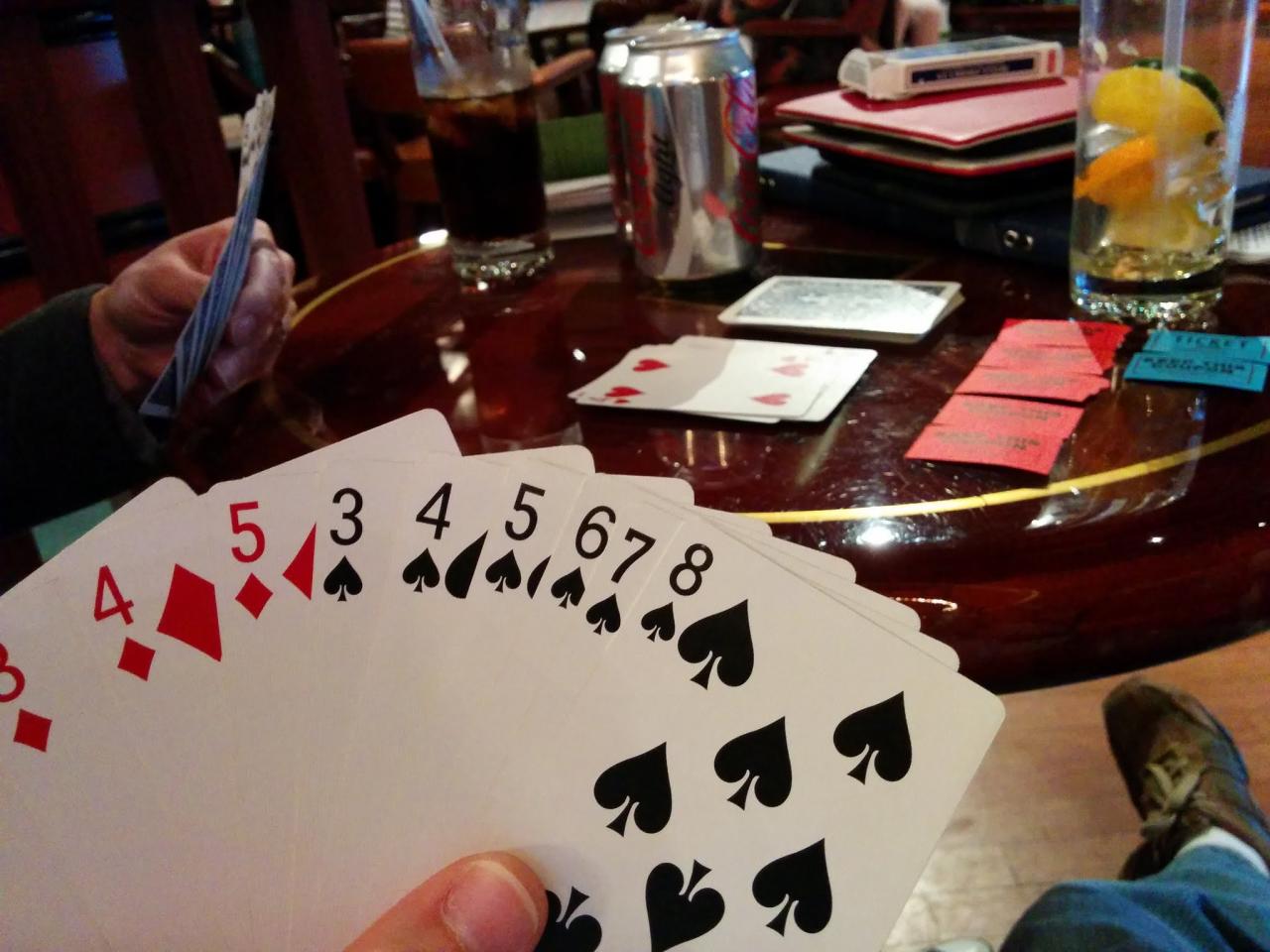A vibrant scene of a card game is captured from the player's point of view. The player holds a hand of cards, revealing combinations of 3, 4, 5 in red diamonds, and 3, 4, 5, 6, 7, 8 in black clubs. Across the table, another player's hand is partially visible, though their cards remain concealed. The tabletop is adorned with two Coca-Cola bottles, an empty glass with fruit pieces, and another glass filled with a dark liquid. Scattered around are several red tickets and two blue tickets. An empty card box rests atop a pile of napkins, and the central game area features two piles of cards. The player's attire is partially visible, showing jeans, white socks, and dark brown tennis shoes. In the background, other groups are also engrossed in their card games, adding to the lively atmosphere of the scene.